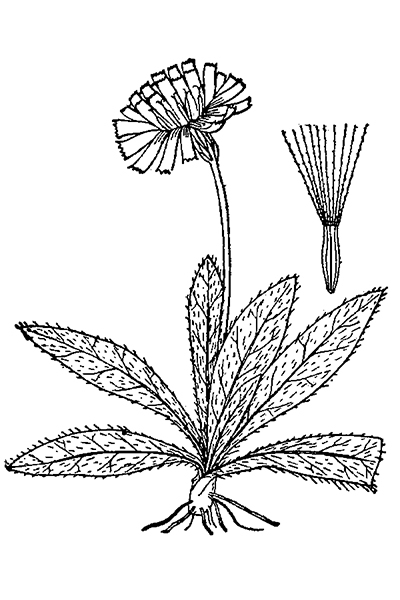This detailed illustration is a black and white line drawing of a single flower, created with a pencil, pen, or possibly computer software, set against a pure white background. The flower features a long, slender stem that extends upward to support many small, rectangular petals. At the base, the stem transitions into a cluster of six pointed, bristly leaves that bear various marks, giving them a somewhat hairy appearance. Below the leaves, the flower's structure continues into a small bulb with roots emanating, suggesting what lies beneath the soil. In the upper right corner of the image, there is an inset showing a segment of the plant, possibly a pollen structure, with spokes radiating from a pointed base. Overall, the illustration combines elements of both above and below ground parts of the plant, capturing a detailed and natural essence.